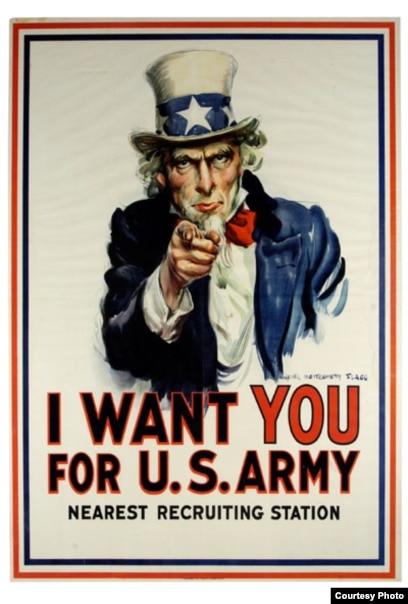This is a color image of the famous World War I "I Want You for U.S. Army" poster featuring Uncle Sam. The poster has a white background framed by a sequence of thin lines in the colors of red, white, and blue, from the outermost to the innermost. Dominating the top of the image is an illustration of Uncle Sam, depicted with curly gray hair, a long white beard and goatee, clad in a distinctively blue jacket with a black collar, a white shirt underneath, and a red bow at his neck. Perched upon his head is a white top hat adorned with a blue band and white stars. Uncle Sam is pointing directly at the viewer, his intense gaze demanding attention. Below him, the bold words "I WANT YOU" are emblazoned, with "YOU" in striking red text outlined in black, and "for the U.S. Army" directly below it in black text outlined in red. Further down, in smaller black text, it reads "Nearest Recruiting Station." In the lower right-hand corner, there is a small black box with white text that says "Courtesy Photo."